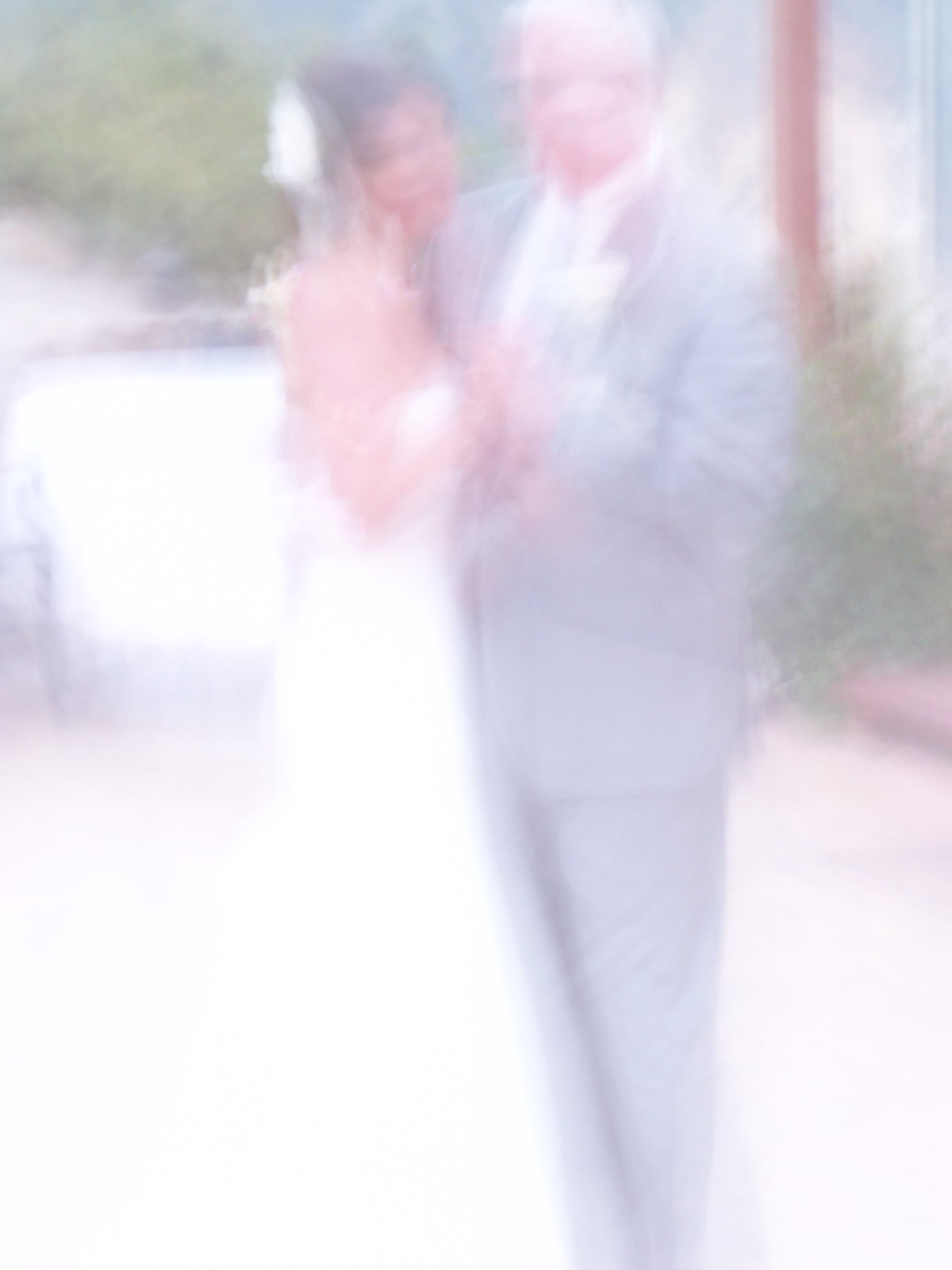This photograph, captured outdoors in harsh, overly bright lighting, is exceedingly blown out and blurred, giving the image an almost painting-like quality. The primary focus is on a couple, presumably at a wedding, though the intense brightness and poor focus obscure specific details. The woman on the left, who has dark hair adorned with a white veil, is dressed in a strapless white bridal gown. However, the bottom portion of her gown is lost in a bright white light, blending into the background. She stands holding hands with a man on her right, who appears older and is dressed in a gray suit with a matching gray necktie. His face, like hers, is difficult to discern due to the blurriness and a peculiar double-vision effect. Surrounding the couple is a murky backdrop featuring indistinct green shrubbery, some bushes in the top left and mid-right corners, a window above the bushes, and a brick area near a sidewalk or walkway to the right. The overall lack of clarity and excessive brightness significantly detract from the detail and focus of the scene.